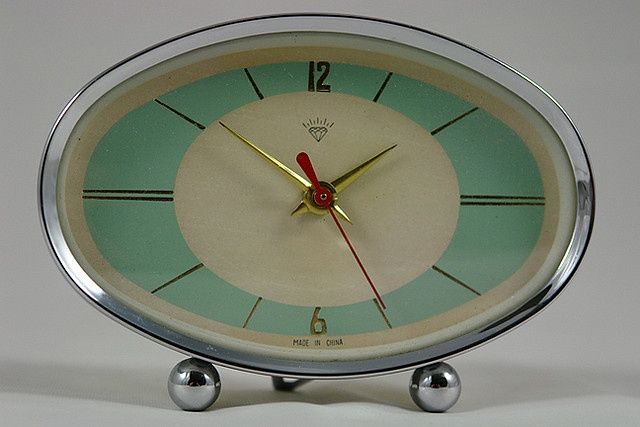This retro oval clock exudes a charming 1950s or 1960s aesthetic, characterized by its chrome and silver outline. It stands gracefully on three round ball feet - two supporting the front and one stabilizing the back. The clock's face, encased in a long oval frame, boasts a delicate blend of light baby blue and off-white hues. A subtle off-white band encircles the outer edges, giving way to a thicker region of baby blue, and culminating in a central circle of pure white.

The time is marked by bold, golden numerals for 12 and 6, while simple lines denote the other hours. Notably, the 3 and 9 are distinguished by double lines. Elegant, pointy gold hour and minute hands sweep across the face, complemented by a slender red second hand. Positioned beneath the 12 is a black-texted diamond emblem, flanked by tiny lines symbolizing shine, and the inscription "Made in China" is neatly printed below the 6.